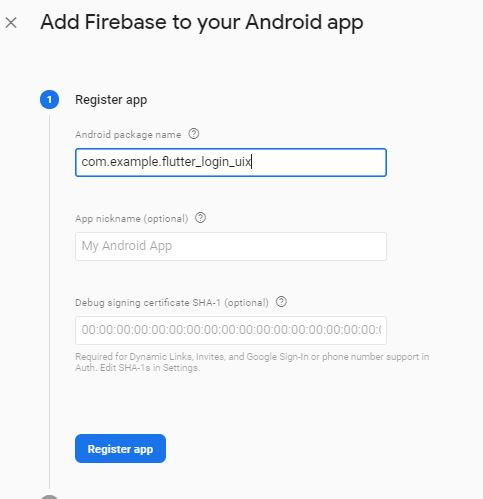The image displays a gray-background interface for adding Firebase to an Android app. In the top left corner, there's a close button marked by an 'X' that allows the user to exit the window. About eighty percent up on the left side of the interface, a blue circle with a white number "1" inside it directs users to "Register app".

Below this indicator, the text "Android package name" appears in small gray font, accompanied by a question mark icon for additional information. Adjacent to this, there's a blue input box pre-filled with "com.example.flutter_login_uix".

Further down in the middle of the page, the label "App nickname (optional)" is displayed in small gray text, also with a question mark for guidance. The corresponding input field is empty but suggests "my Android app" as a default nickname.

Continuing downward, the interface specifies "Debug signing certificate SHA-1 (optional)" with an accompanying question mark. This field is filled with repeating "00:00:00:", indicating where the certificate information should be entered. Below the input box, a note in gray text indicates that the SHA-1 is required for features like dynamic links, Google sign-in, and phone number support in authentication. It also mentions that SHA-1 can be edited in settings.

At the bottom right corner of the window, there's a blue button with white text that reads "Register app," inviting users to complete the registration process.